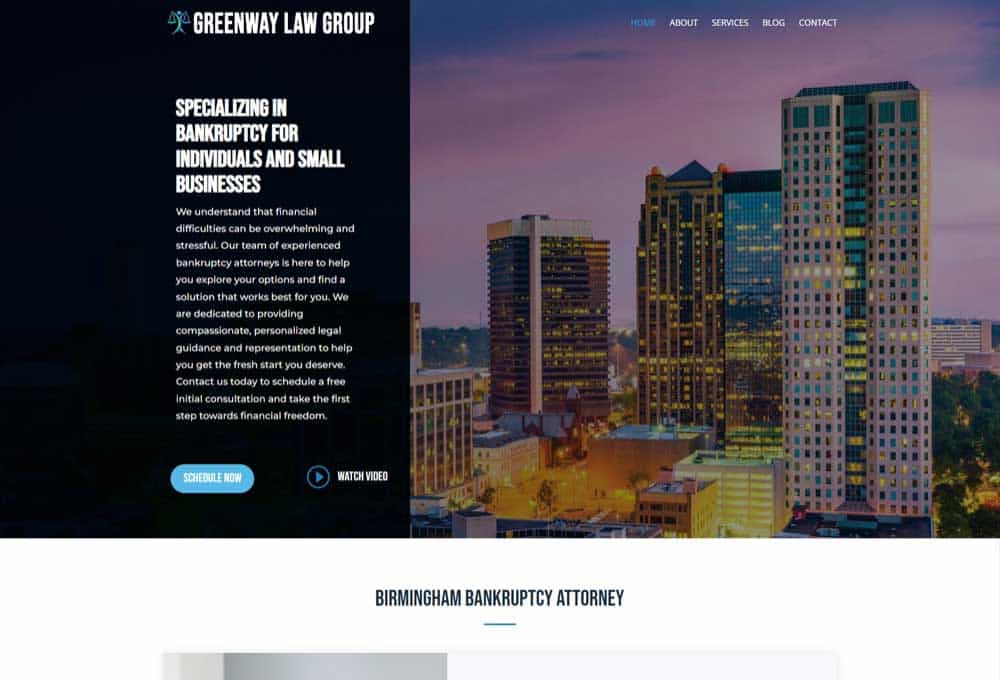The image depicts the homepage of a law firm's website. The layout is landscape-oriented, optimized for viewing on larger screens like computers or horizontally-aligned tablets. A black vertical rectangle occupies the left third of the screen, featuring the header "Greenway Law Group" in white text, accompanied by a blue logo of a figure holding scales at the top. Below the firm’s name, the text "Specializing in Bankruptcy for Individuals and Small Businesses" is prominently displayed in white. Beneath this tagline, there is a block of descriptive text, followed by two actionable buttons: "Schedule Now" and "Watch Video."

The remaining two-thirds of the screen showcases a scenic view of a city, likely Birmingham—though it's ambiguous whether it's Birmingham, Alabama, or Birmingham, England. The cityscape features various high-rise buildings illuminated by city lights. This image has a dark, possibly purple overlay that mutes the brightness.

At the bottom of the main image, a horizontal black bar contains the text "Birmingham Bankruptcy Attorney" in white, separated by a thin horizontal line. A gray rectangle at the bottom of the page rounds off the design, possibly housing additional navigational or informational elements.